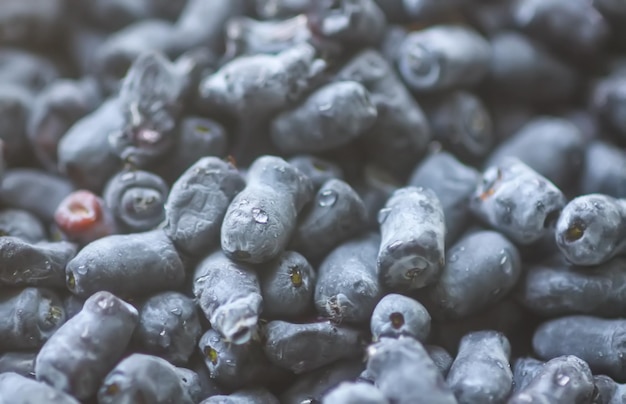This horizontal, rectangular image portrays a large, scattered pile of oblong, cylindrical objects that are predominantly dark blue-gray, somewhat resembling the color of blueberries. However, their shape and surface texture suggest they are not fruit but rather some kind of inorganic material, potentially small stones or pellets used in a fire pit. Some of these objects have a whitish, powdery surface while others are simply dark blue-gray. A contrasting feature is a solitary red object on the left side, which may be part of the same material but in a different color. The image's foreground reflects light, indicating metallic or wet surfaces, while the background fades into a blur, emphasizing the endlessness of the pile. There is also a slight suggestion of organic material at the tips of some pellets, adding an element of ambiguity to their true nature. The overall scene is punctuated by water droplets, giving the appearance of dampness throughout.